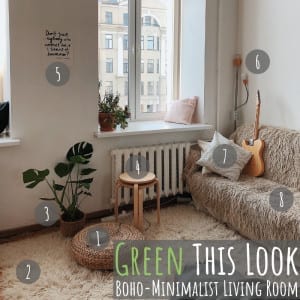This detailed photograph showcases a serene and calming boho minimalist living room, as indicated by the text at the bottom right that says, "green this look, Boho Minimalist Living Room." The room is bathed in light, revealing a high-up setting, possibly in a condo, as one can see several floors up through the window. The decor features a beige and light color palette, except for the two vibrant green plants that add a touch of nature.

A furry-textured couch is positioned on the right side of the image, adorned with two pillows and a guitar. Directly beside the couch is a small stool and a radiator against a white wall. A large, shaggy rug covers the floor, adding to the room’s cozy, tactile aesthetic. Several objects in the room are labeled with gray circles and white numbers, suggesting an interactive guide possibly for a website like Pinterest.

Additional furnishings include a small round stacking table and a wicker floor seat, enhancing the bohemian vibe. The window sill is spacious and styled with a pillow and a potted plant, creating a cozy nook. Yet another plant with green leaves sits against the wall in a brown pot. The numbered tags extend to a small note on the wall next to an item marked as number 5.

Overall, the living room's combination of eclectic decor, soft textures, and natural elements creates an inviting and peaceful atmosphere.